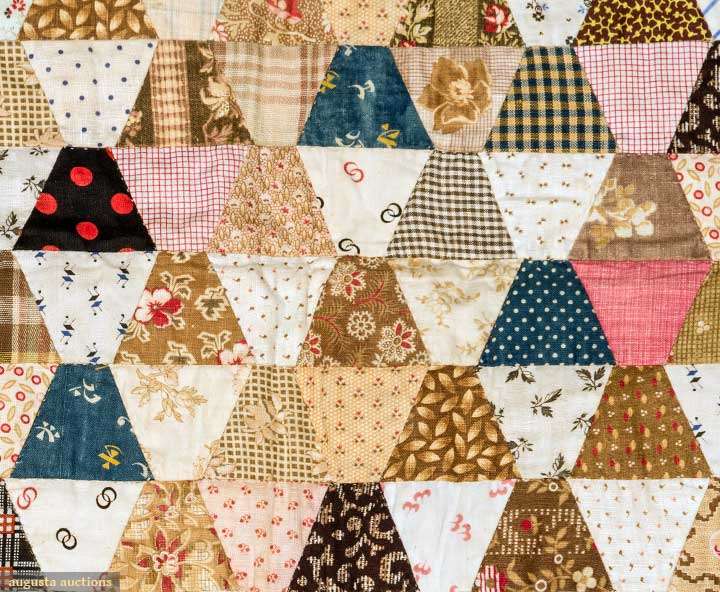The color photograph, taken in a landscape orientation, showcases a meticulously crafted vintage patchwork quilt. This homemade quilt features intricate patterns and vibrant colors that extend seamlessly from top to bottom and left to right. The dominant colors include dark brown, dark blue, cream, and pink, contributing to its richly detailed aesthetic. 

The quilt comprises about 12 rows of designs, partially cut off at the top. Each row primarily consists of alternating triangles forming hexagonal shapes. Meanwhile, we observe approximately six rows of rectangles, with five fully visible and a sixth row partially cut off. Various intricate patterns traverse these rows, including a motif of peanuts on a brown background, paw prints in brown on a light background, brown with yellow stars and white dots, red crisscross lines over white, and white with red and blue eights or S shapes.

Additionally, the quilt features designs with butterflies, a black pattern accentuated with gold, and several floral patterns that intersect each other. On the bottom left corner of the image, in small yellow font over a clear border, the text reads "The Gusto Auctions." This detailed and vibrant quilt exemplifies the style of photographic representationalism, capturing its textures and patterns with realism.